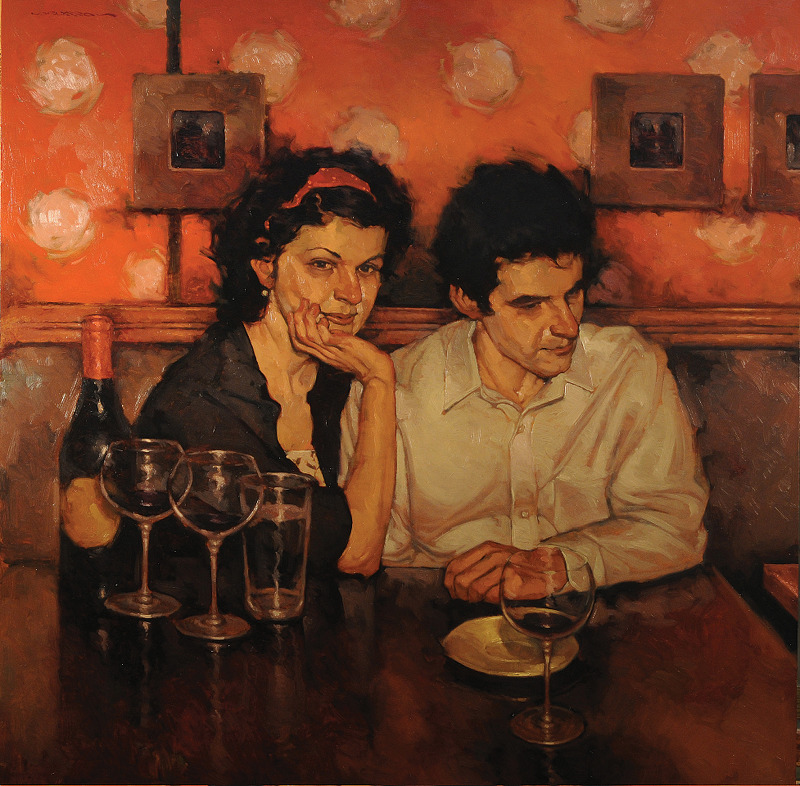The painting, likely done in a classic oil-on-canvas style, displays a man and a woman seated at a table in what appears to be a restaurant or patisserie. The background showcases an orange wallpaper with white polka dots, adorned with multiple brown-framed pictures. The lower part of the wall, separated by a brown trim, is painted gray. In front of the subjects is a dark brown reflective table, where several items are meticulously placed: a blue and black wine bottle with a white label and red top, three wine glasses assumed to hold red wine, a nearly full water glass, and a saucer that resembles an ashtray but is empty.

The woman, positioned on the left, has short dark curly hair pulled back with a red headband. She is adorned with small pearl earrings and is dressed in a black blouse over a white shirt. Her dark eyes suggest contemplation as she rests her right hand thoughtfully against her chin. She leans closely towards the man beside her, almost clinging to him. The man, on the right, gazes downward and away, his expression tinged with sadness. He sports dark curly hair and wears an off-white long-sleeved button-up shirt. The pair's composition, set amid the cozy yet somber ambiance of their surroundings, evokes a scene rich with unspoken emotions and subtle tension.